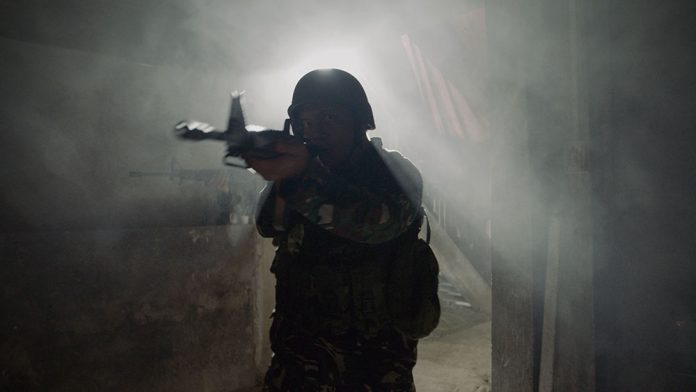The horizontally aligned rectangular image captures a scene that appears to be from a realistic video game, depicting a soldier in a dark, smoky environment. The soldier is centrally positioned, facing the camera with a determined look. He has a green helmet on and is clad in a camouflage uniform with black tactical gear, including a bag on his back. His rifle is held in a ready position, aimed forward with both hands, indicating he is prepared for imminent action. The background reveals the inside of a building with stone walls and what seems to be a concrete floor. Smoke, potentially from a recent gun battle, envelops the scene, adding to the chaotic atmosphere. A doorway and a set of stairs are visible in the blurred, smoky background, suggesting the soldier is about to enter another part of the building. The combination of these elements creates a tense and immersive moment, as if the soldier is emerging from a recent skirmish, ready for the next confrontation.